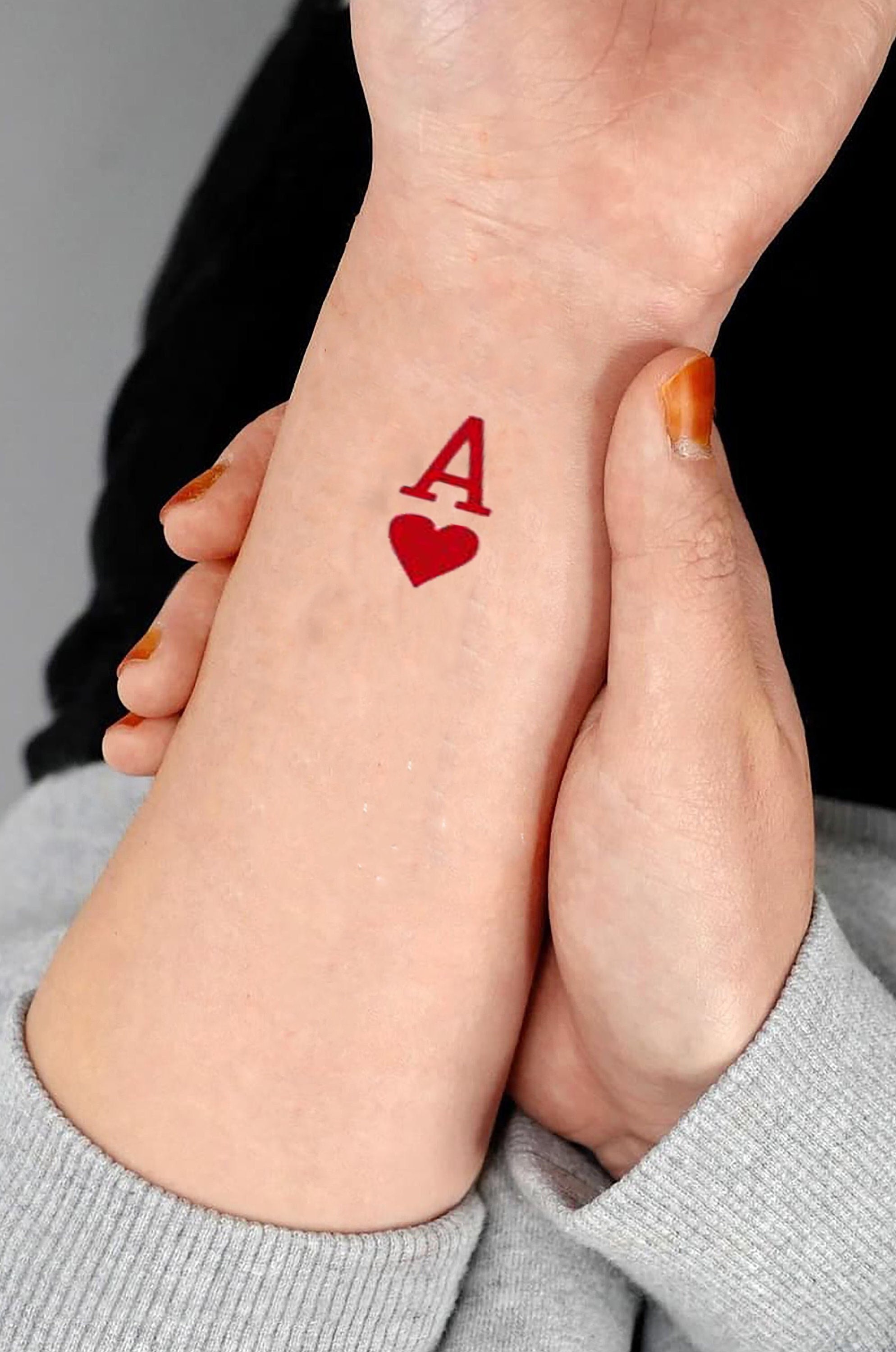In this detailed image, a young white woman proudly displays her wrist tattoo, prominently featuring a stylized Ace of Hearts. The tattoo, on the inner part of her wrist just below her hand, showcases a block-letter 'A' in red with a small heart underneath, both elements being of significant size. Her clear, well-hydrated skin enhances the tattoo's vividness, while her red nail polish accentuates its design. She wears a long-sleeve sweatshirt with ribbed cuffs, drawing extra attention to her wrist. The background reveals a hint of another person or a piece of dark cloth, adding a subtle layer of intrigue to the scene.